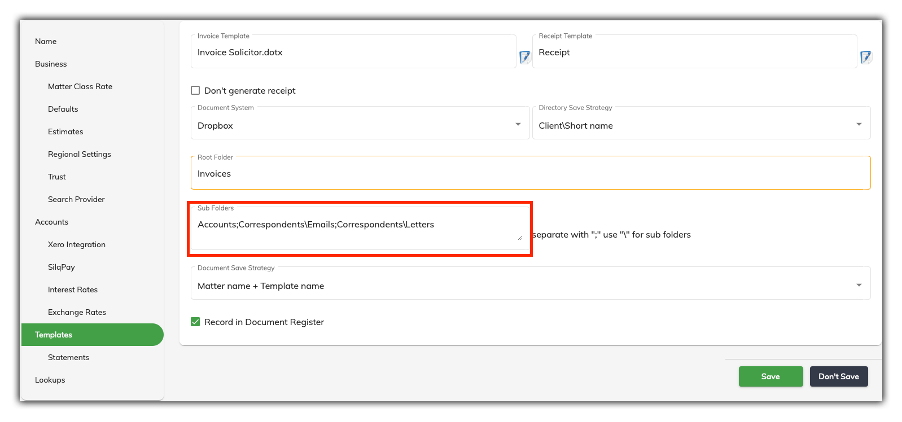The image is a screenshot of a computer page, likely viewed on a laptop or desktop, presented in a rectangular format. It features a vertical column on the left with a light gray background and black text. At the top of this column, headings are clearly listed: "Name," "Business," "Matter," "Class Rate," and "Defaults." Following these are additional categories: "Estimates," "Regional Settings," "Trust," "Search Provider," and then another header labeled "Accounts." Beneath "Accounts," the text is somewhat hard to read, but it appears to mention "Integration," with the subsequent items possibly being "Skip Pay," "Interest Rates," and "Exchange Rate."

On the right side of the page, which has a white background, there are various drop-down menus and options available for user interaction. One of the drop-down menus includes an option for "Client Short Name." Another drop-down menu appears to be related to receipts. There is also a checkbox labeled "Don't Generate Receipt," allowing users to opt-out of receipt generation. Notably, a red rectangular box is highlighting another section of the page, drawing attention to a specific area for further interaction or editing.